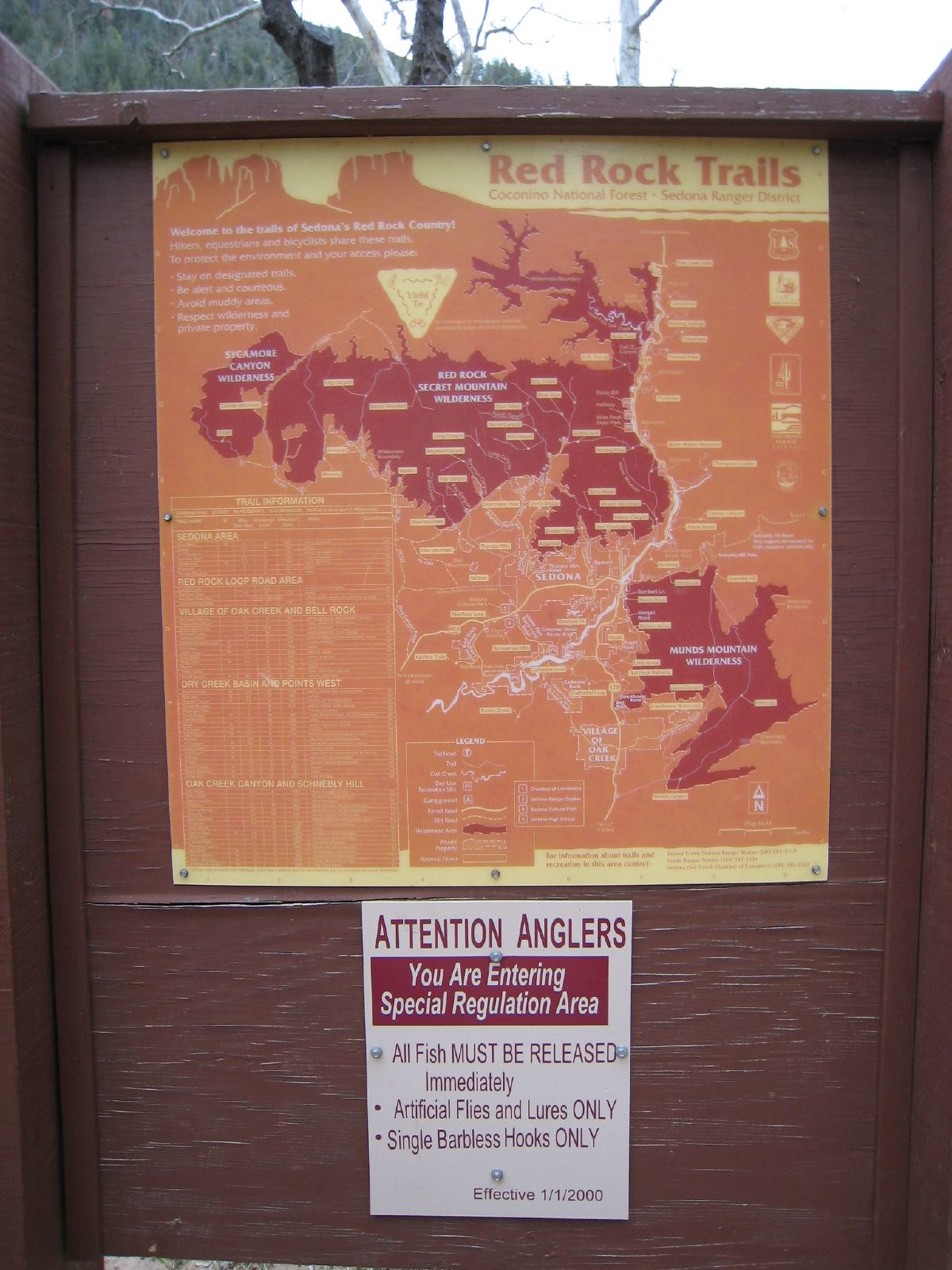The weathered wooden signboard, painted brown but revealing gray and dark patches underneath due to chipping and cracking paint, stands prominently. It hosts a large, vividly colored map of the Red Rock Trails, specifically depicting the Sedona and Red Rock Secret Mountain Wilderness areas. The map, dominated by shades of orange, yellow, and red, illustrates various regions of wilderness, lakes, and rivers. Trail markings are shown in white, with specific parts labeled in yellow. A comprehensive table of trail information occupies the bottom left corner, also colored in yellow, though its text remains too small to decipher in detail. Below the map, a smaller white sign is affixed with screws, bearing a crucial warning in red text: "ATTENTION ANGLERS YOU ARE ENTERING A SPECIAL REGULATION AREA. ALL FISH MUST BE RELEASED IMMEDIATELY. ARTIFICIAL FLIES AND LURES ONLY. SINGLE BARBLESS HOOKS ONLY. EFFECTIVE 1.1.2000." This signage indicates specific fishing regulations within the national forest area.